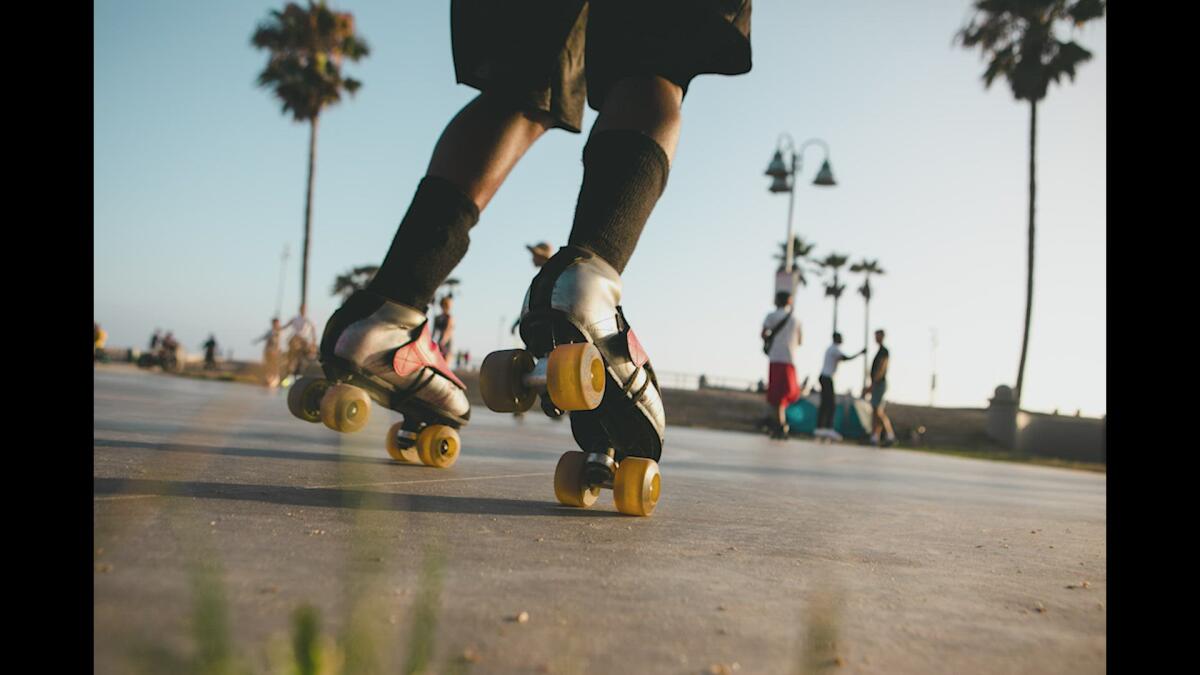The photograph, captured at ground level in the early evening sun, shows the bottom half of a person roller skating on a parking lot. The focus is on their white roller skates, which feature yellowing wheels and black straps. The skater is wearing green socks paired with olive green jean shorts. The right skate is lifted, with the toe pointed down, suggesting movement, while the left skate is similarly off the ground but not as elevated. The backdrop includes lines on the roadway, several palm trees, and lamp posts. Blades of green grass appear blurry in the foreground, adding depth to the image. In the distant background, there's a group scene: three people near a light post, two of whom seem to be in a heated conversation, while another approaches them with a crossbody bag. Scattered further back, more individuals can be seen, indistinct but adding to the bustling atmosphere of what seems to be a popular skating spot.